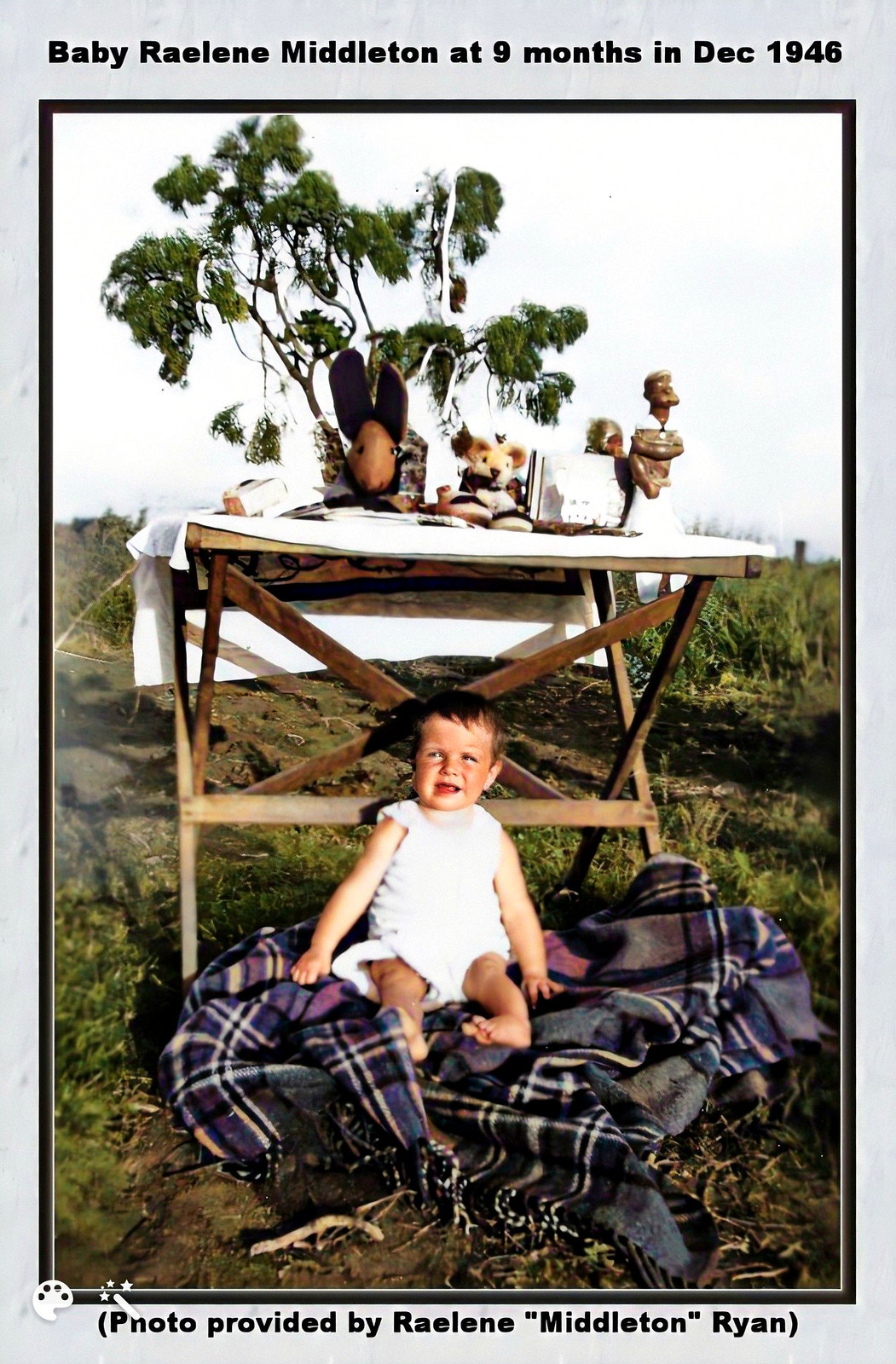The photograph shows a baby, approximately nine months old, identified as Baby Raleigh Middleton, from December 1946. The image is framed with a thin black line within a gray border. The top border contains black text that reads, "Baby Raleigh in Middleton at nine months in December 1946," while the bottom border states, "Photo provided by Raleigh in Middleton Ryan." The baby, with brown hair, is dressed in a white outfit and is sitting on a blue and purple plaid blanket spread across a grassy hillside. Behind the child is a foldable wooden table covered with a white tablecloth, which holds a couple of books, a stuffed rabbit, a stuffed mouse, and a wooden carving. In the backdrop, lush greenery and a tree can be seen.